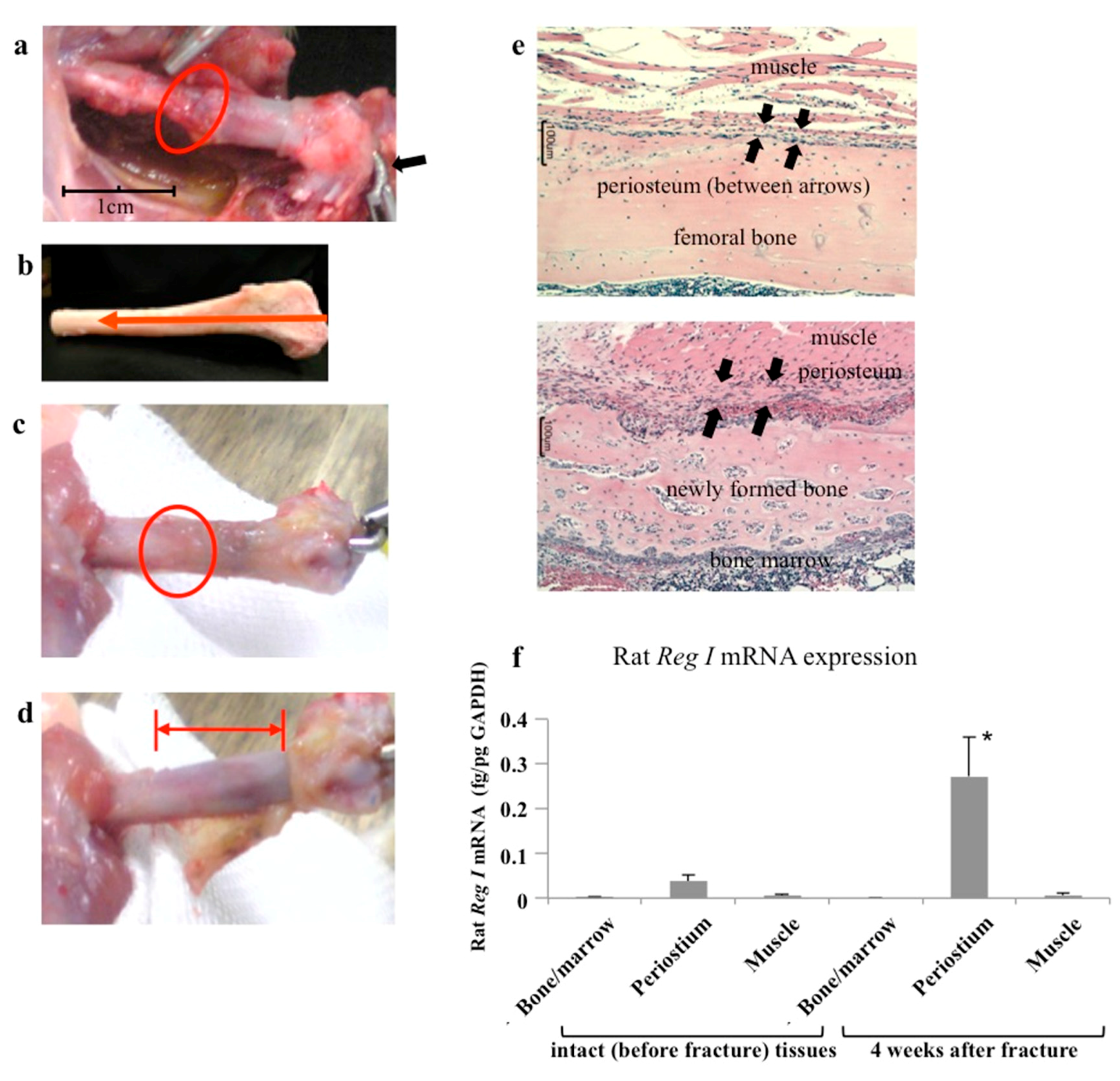The image set details a step-by-step medical procedure involving a femoral bone and its surrounding muscle tissues, with the pictures labeled A through D on the left and E to the right. Image A displays a bone where a section has been carved, delineating a separation from the muscle tissue. A red circle highlights this specific area. Image B reveals an old, cleaned bone with an arrow pointing downward on its left side. In Image C, the bone is extracted from the body, with a red circle indicating another specific area of interest. For Image D, the bone appears further stripped, with two arrows pointing to distinct walls. The right-most section, labeled E, features annotations specifying various anatomical and experimental elements: "muscle, periosteum between arrows, femoral bone," and highlights "muscle periosteum, newly formed bone, bone marrow, RAT Reg 1 mRNA expression."

There is also a graph situated at the bottom right, marked with vertical axis numbers (0.1, 0.2, 0.3). It details "RAT Reg 1 mRNA expression," showing values of "FG over PG, GAPDH." The graph compares bone marrow, periosteum, and muscle at two different stages: intact tissues before fracture and four weeks post-fracture, indicating notable differences in mRNA expression levels.